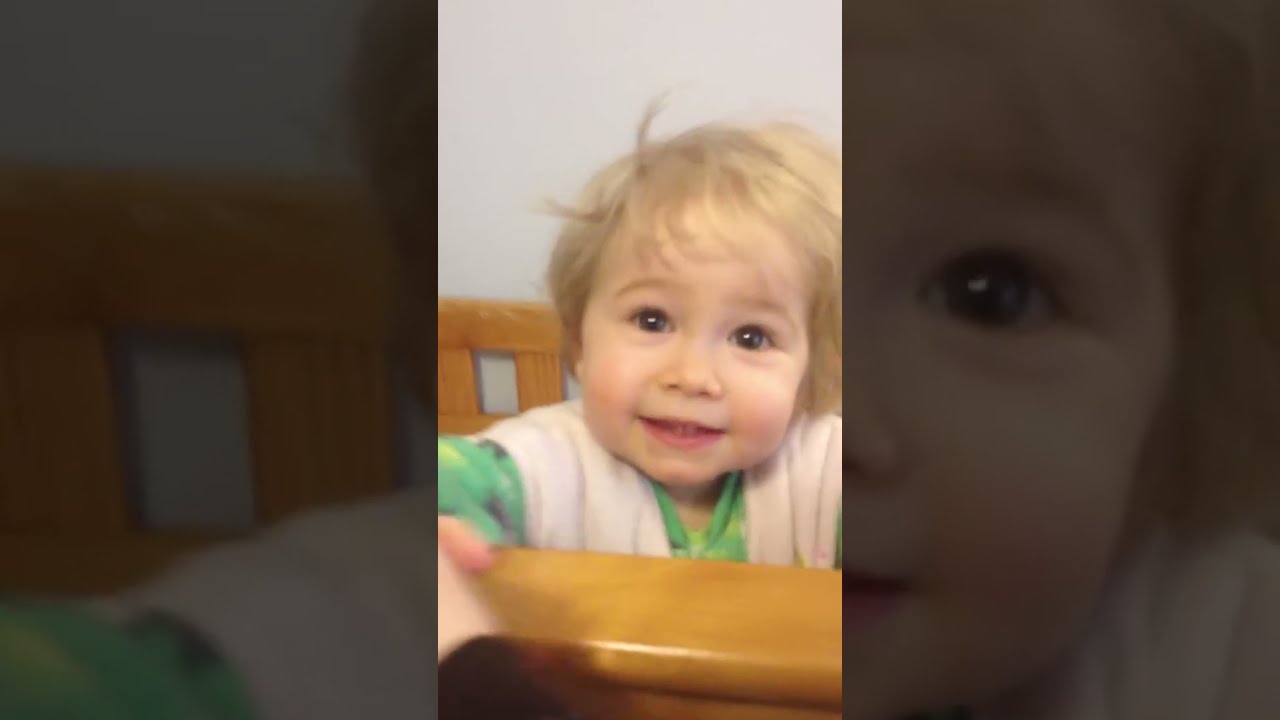The image displays a baby standing in a wooden crib, centered in the frame, with a white wall as the backdrop. The baby, possibly a boy or girl, has striking blonde hair that is slightly messy, and large, beady blue or brown eyes. The baby's face is chubby with slightly red cheeks, giving a well-fed appearance. Dressed in a white onesie with a green sleeve, the child is holding onto the crib's wooden railing for support, suggesting recent mastery of standing up. Inside the crib is a pink, knitted blanket, visible through its weaved holes. The crib itself is light brown, constructed with vertical wooden slats. The scene is well-lit, indicating an indoor setting. The overall vibe is that of a cozy, standard room for a young child.